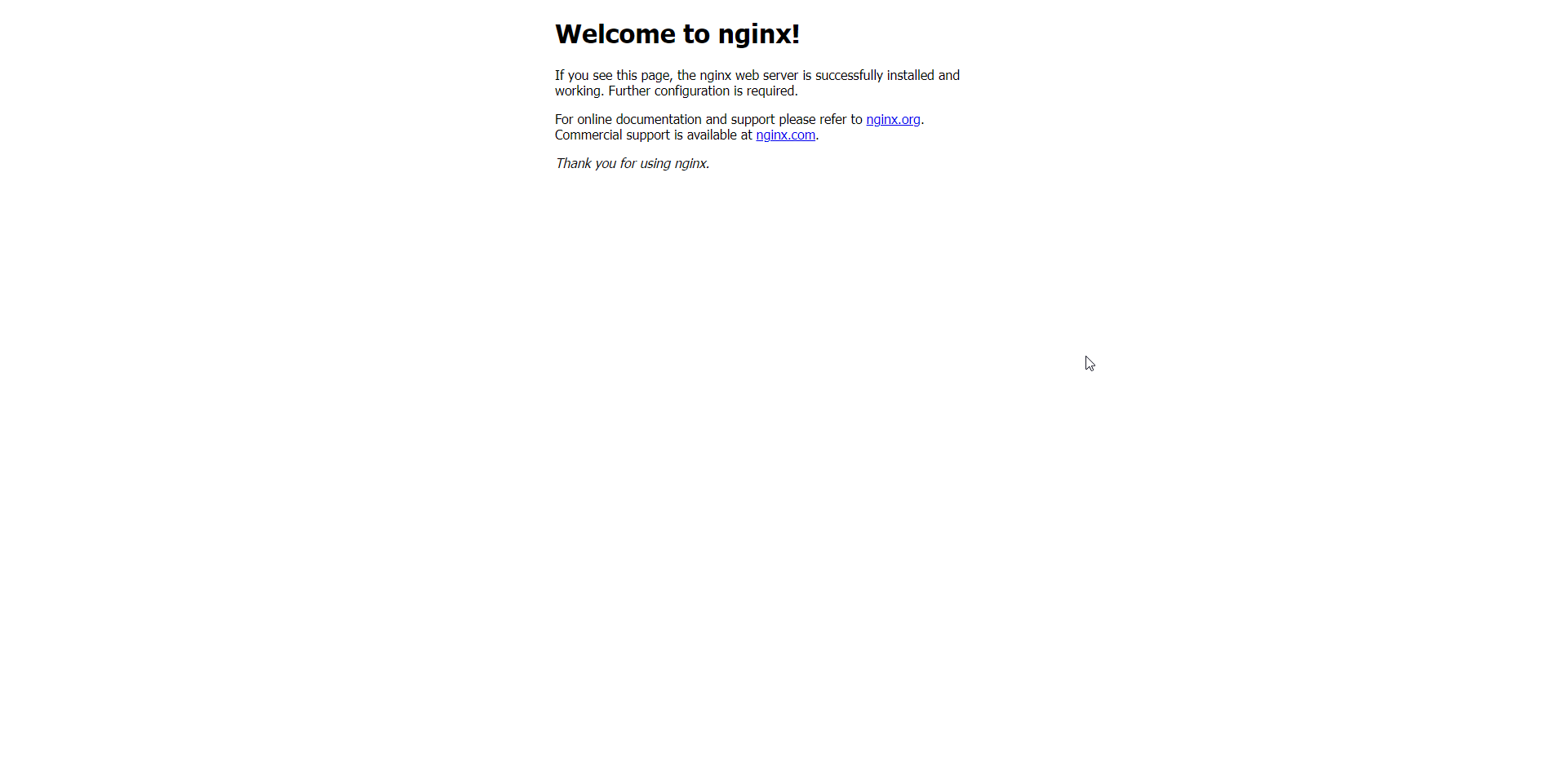The image features prominently centered text with URLs at the top and a white mouse pointer towards the bottom right corner. The URLs, "nginx.com" and "nginx.org," are underlined and displayed in blue. The main text, written in black, reads: "Welcome to NGINX". This welcome message is bold. Beneath it, the text continues: "If you see this page, the NGINX web server is successfully installed and working. Further configuration is required. For online documentation and support, please refer to nginx.org. Commercial support is available at nginx.com". The image concludes with a note of gratitude: "Thank you for using NGINX". The URLs "nginx.org" and "nginx.com" are the only blue text, emphasizing their importance for further resources and support.